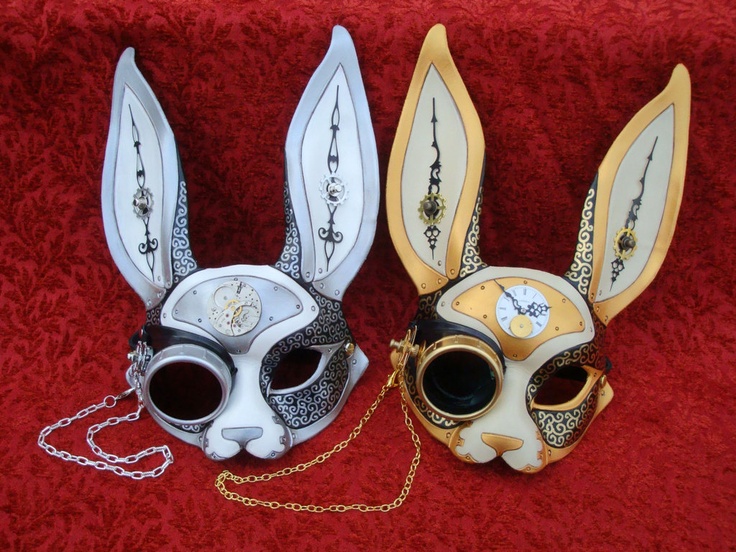The image showcases two ornate and intriguing masks placed against a richly textured red cloth background that features a subtle leaf pattern. The mask on the left is silver, while the one on the right is golden. Both masks have intricately designed, large, round eye openings paired with a cat-like eye on the right side, each outlined in their respective metal color—gold for the gold mask and silver for the silver mask.

Each mask is adorned with a small clock on the forehead, with the golden mask's clock displaying the time "five to three." Adding to their elaborate design, each mask features two prominent, upward-facing "ears" that suggest an anthropomorphic rabbit or hare, further embellished with what appears to be clock hands inside.

A chain is attached to the left side of the silver mask and the right side of the gold mask, positioned in a way that would correspond to the right side if worn on a face. These fascinating, Baroque-style masks evoke a sense of mystery and intrigue, reminiscent of masquerade balls and secretive gatherings.